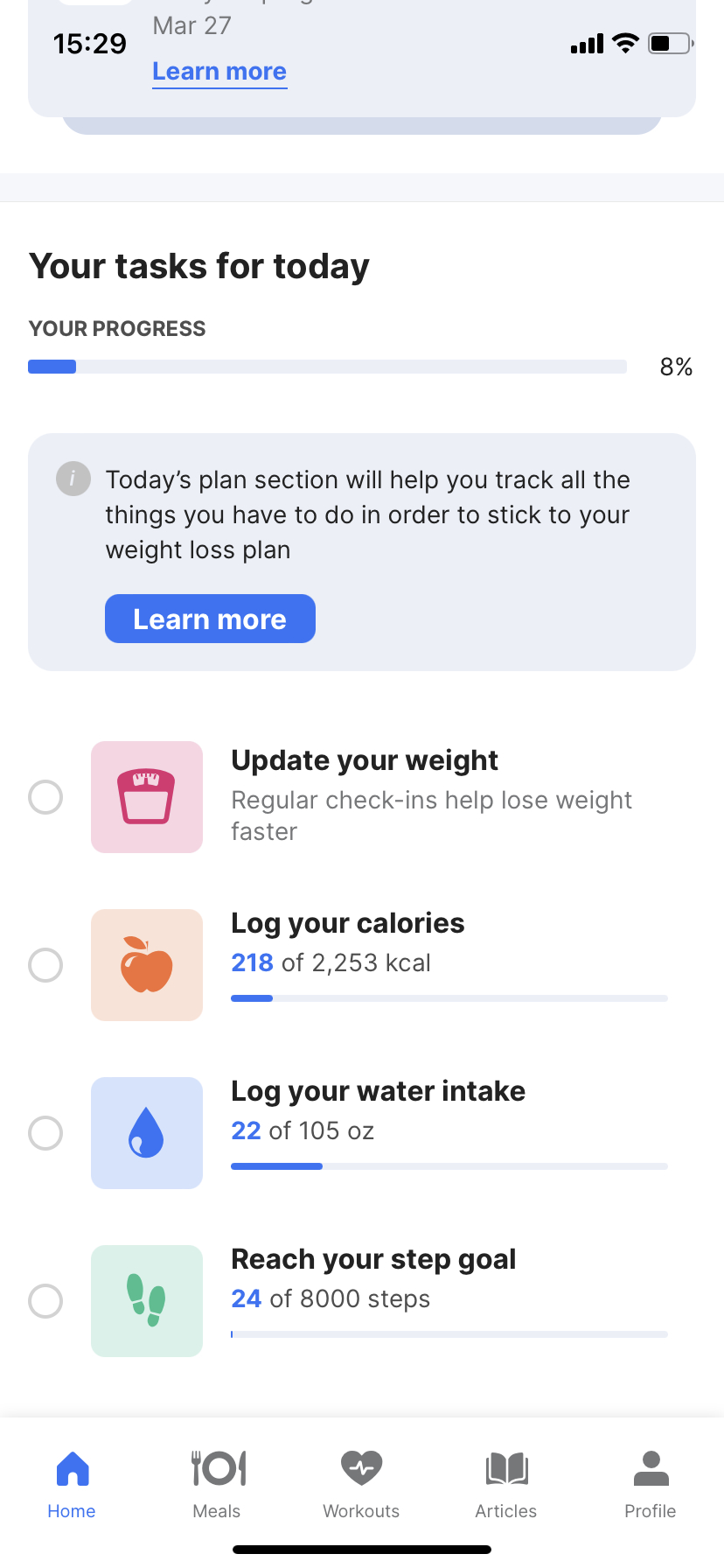**Caption:**

A detailed screenshot from a mobile phone app displays a comprehensive weight loss tracking dashboard. The title "Your Task for Today" is prominently shown at the top on a white background with bold black text. Directly beneath the title is an 8% complete progress bar, colored in blue. Below this progress bar, a transparent gray box provides guidance with the text: "Today's plan section will help you track all the things you have to do in order to stick to your weight loss plan." A blue "Learn More" button is situated below this informative text.

Following the gray information bubble, four task items are listed, each with a circular checkbox next to them. 

1. The first task, "Update your weight," is represented with a scale icon on a pink background.
2. The second task, "Log your calories," features an orange apple icon and displays a specific progress bar showing 218 out of 2,253 calories logged.
3. The third task, "Log your water intake," is illustrated with a blue water droplet icon and a progress bar indicating 22 out of 105 ounces logged.
4. The final task, "Reach your step goal," includes green footprints and displays a progress bar showing 24 out of 8,000 steps completed.

At the bottom of the screen, a navigation bar contains five icons for easy access: Home, Meals, Workouts, Articles, and Profile.